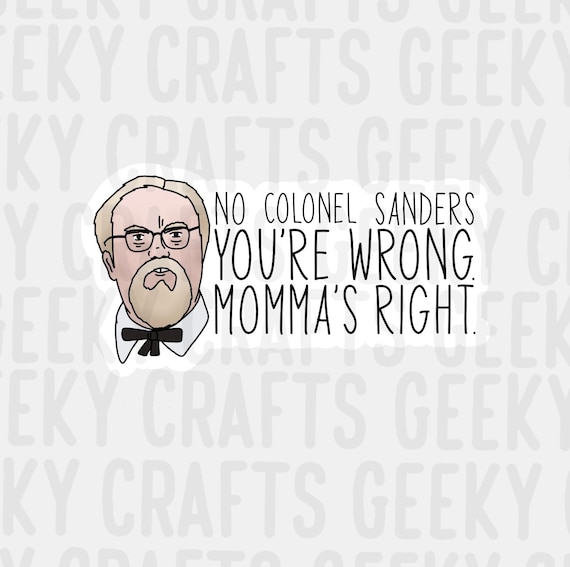The image portrays an advertisement, featuring a light gray square background repeatedly overlaid with the words "Geeky Crafts" in a slightly darker gray. At the center of this backdrop is an animated depiction of Colonel Sanders, distinguishable by his white hair, beard, glasses, and characteristic black bow tie over a light blue collar. He appears to be frowning subtly, adding to the humorous tone. To his right within a white, rectangular outline are the words "No, Colonel Sanders, you're wrong, mama's right," serving as a playful and amusing caption. The overall image is designed to provide humor and appeal to fans of "Geeky Crafts."